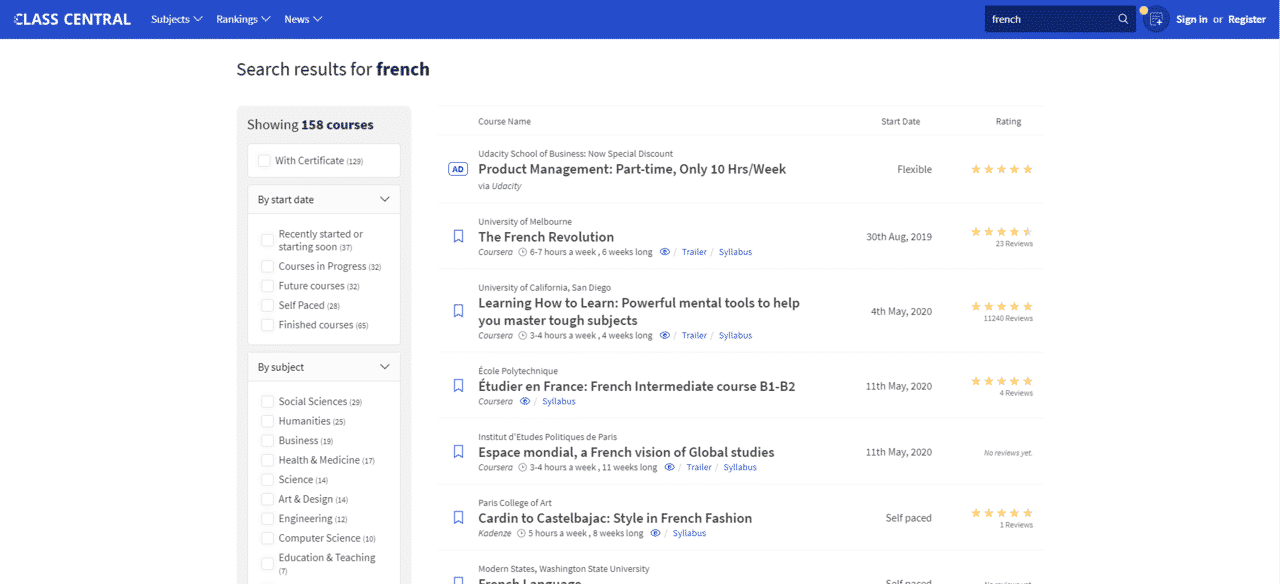The screenshot displays the webpage of 'Class Central,' identifiable by the blue navigation bar at the top with white text. The bar includes 'Class Central' on the left and three drop-down menu options labeled 'Subjects,' 'Rankings,' and 'News.' On the right side of the bar, there is a search field with the word 'French' entered, and options to 'Sign In' or 'Register.'

Below the navigation bar, a vertical column on the left shows the text 'Search Results for French,' indicating a total of 158 courses found. Adjacent to this column is a list of the search results, each including course titles and brief information.

Among the courses listed are:
- 'Product Management' (part-time)
- 'French Revolution'
- 'Learning How to Learn: Powerful Mental Tools to Help You Master Tough Subjects'
- 'Étudier in France,'
- 'Espace Mondial: A French Vision of Global Studies'
- 'Carden to Castelbaja: A Style in French Fashion'

To the right of the course titles, columns indicate the start dates and user ratings with accompanying stars. The bottom part of the screenshot is cut off, preventing a full view of the complete list of courses.